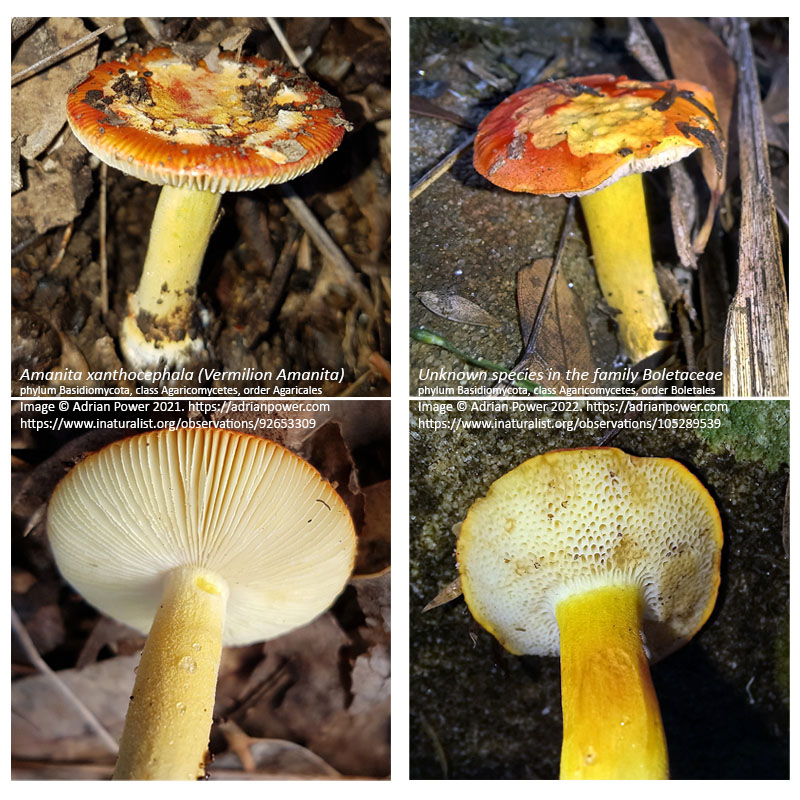In this composite image, there are four photos of mushrooms arranged in a grid. The top left image captures a top-down view of a mushroom labeled "Amanita xanthocephala (Vermilion Amanita)," displaying a striking reddish-orange cap with visible damage, such as missing chunks potentially caused by bugs. The bottom left photo reveals the underside of this mushroom, showcasing its gills. Both of these images feature a text overlay attributing the photos to Adrian Power, with a copyright notice for 2021 and links to his website and an iNaturalist observation page.

The top right image depicts another mushroom, this time an unknown species within the Boletaceae family. It similarly has a reddish-orange cap with missing chunks, and the label includes its classification: phylum Placidiomycota, class Agaricallis, and order Boletalis. The bottom right image provides a view of the underside of this mushroom, again revealing its gills. This image also includes Adrian Power’s copyright information and associated links.

All four photos share a similar aesthetic with dirty-looking backgrounds, possibly highlighting their natural habitat. The mushrooms in both sets display yellow stems with white undersides, despite the differing classifications.